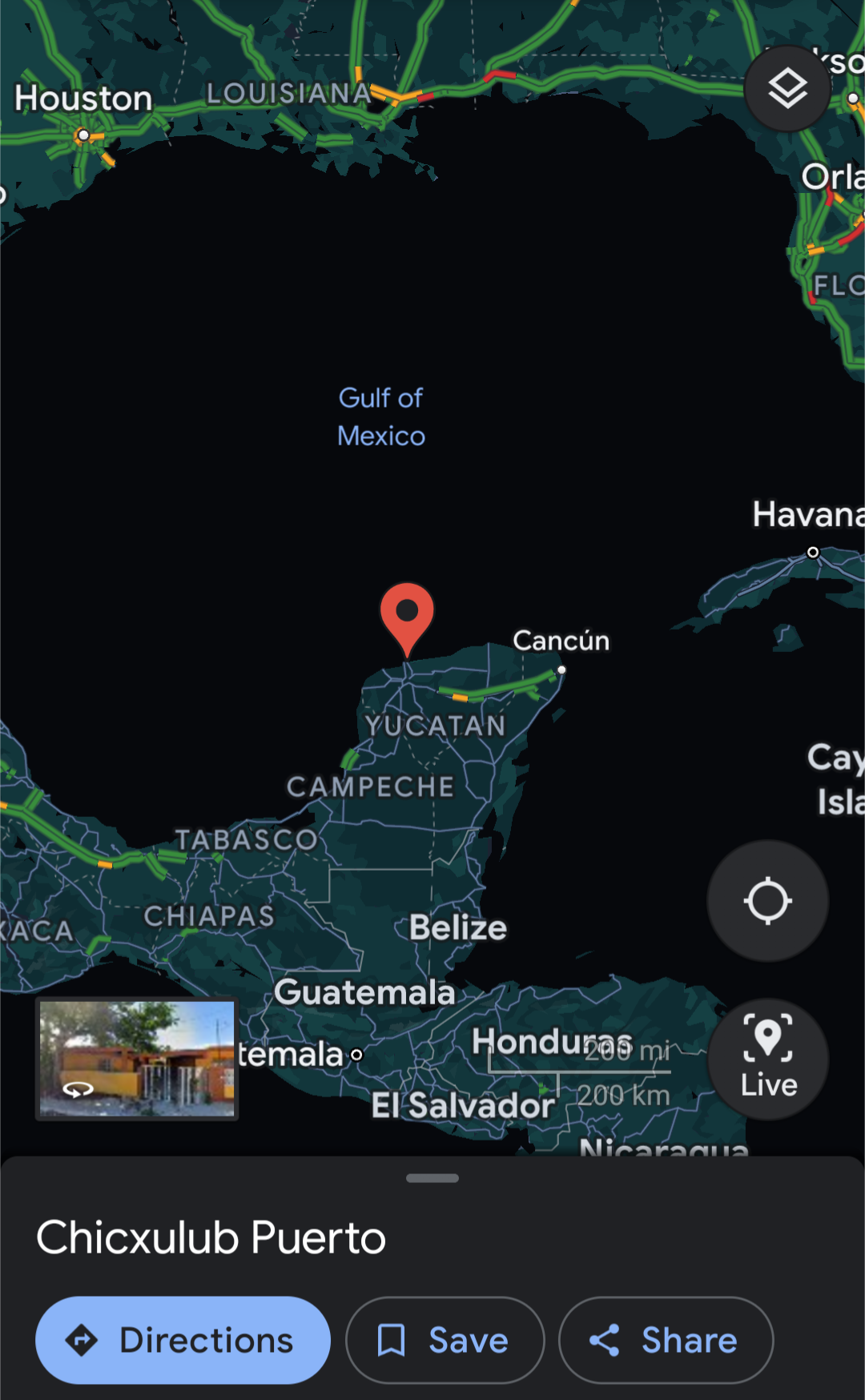The image is a vertically rectangular screenshot captured from a cell phone. Occupying the majority of the frame is a detailed map that prominently features the Yucatán Peninsula and the Gulf of Mexico. Near the top-center of the map, a pin is specifically placed above the Yucatán region, indicating a location of interest. At the bottom of the image, a black, vertically rectangular banner is overlaid, providing additional information. In this banner, directly beneath the pinpointed map location, the text spells out "CHICXULUB PUERTO" in clear lettering. Further down, the banner showcases three clickable buttons designed for user interaction. The button on the left is light blue with black text reading "Directions." To its right are two black buttons with blue text, labeled "Save" and "Share," respectively.